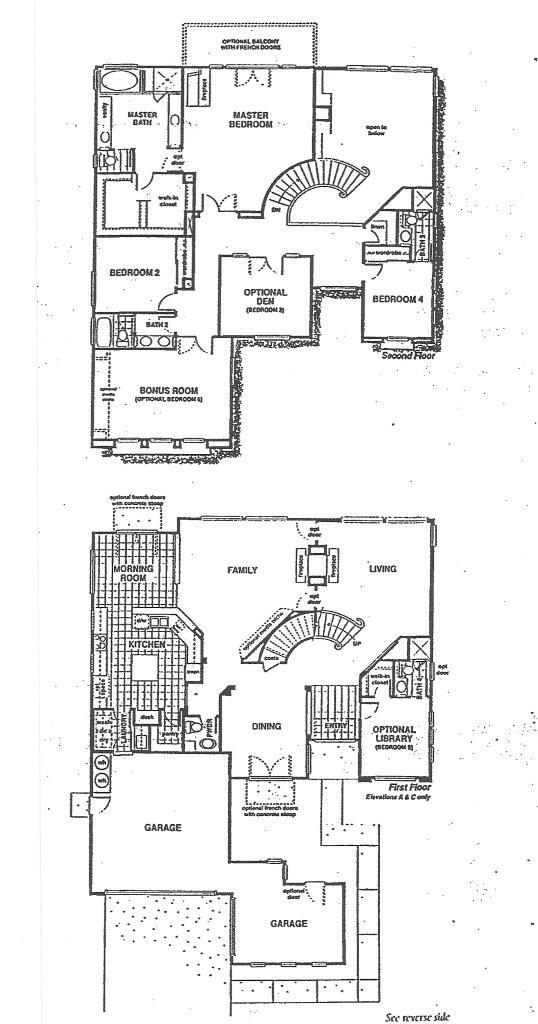This set of black and white floor plans provides an intricate layout of a two-story home, complete with detailed descriptions of each area. 

The first image depicts the second floor, featuring a master bedroom complemented by a luxurious master bath. A dramatic Cinderella-style staircase elegantly wraps around near the foyer, suggesting cathedral ceilings and an open area below. Adjacent to the staircase is an optional den, adding flexibility to the floor plan. Bedrooms 2 and 4 are also shown, connected by a hallway that leads to a bonus room located near Bedroom 2, offering additional living space or a potential office.

The second image illustrates the first floor layout. At its heart, a family room and a living room are seamlessly connected by the same Cinderella staircase, emphasizing the home's grandeur. Off the kitchen is a quaint morning room, likely intended as an eating nook, characterized by a series of squares marking the kitchen counters and island. This design demonstrates the flow from the kitchen to the dining area. Additionally, the plan includes an optional library and another labeled room, possibly denoting an entry area. The layout also identifies a notable feature of two diagonally connected garages, enhancing both convenience and storage options for the home.